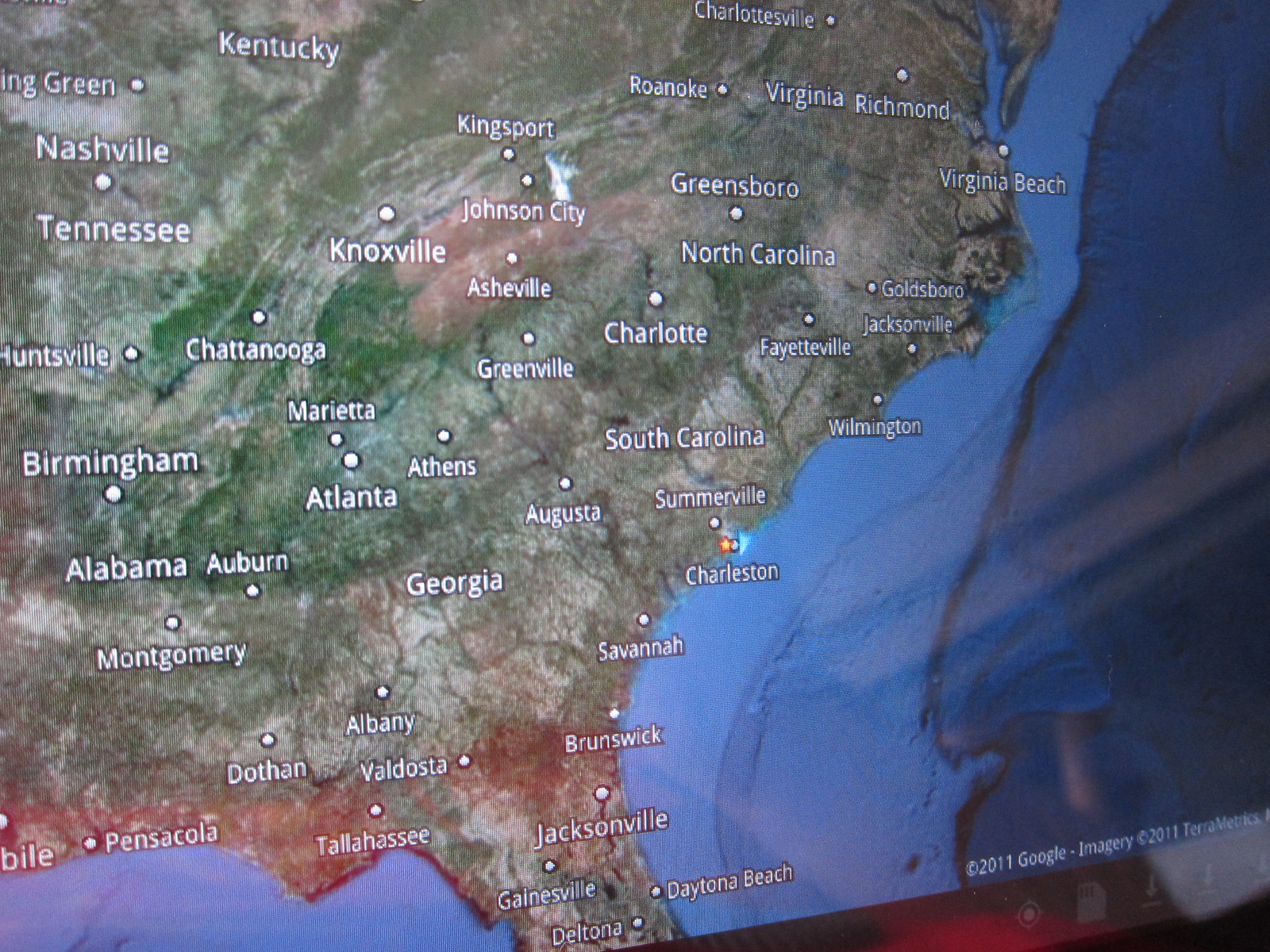This detailed image depicts a computer screen showing a zoomed-in map of the southeastern United States, extending from Virginia to Daytona Beach, Florida, and from Kentucky to Mobile, Alabama. The map showcases topographical features, including rivers and varied terrain, with green areas indicating vegetated regions and brown areas representing less lush landscapes. Major and mid-sized cities such as Charlottesville, Virginia; Nashville, Tennessee; and Huntsville, Alabama are labeled in white. The Atlantic Ocean, to the right of the map, transitions from light blue near the shore to darker blue further out. The map is marked with "Copyright 2011 Google" and "Copyright 2011 Terrametrics" in the bottom right-hand corner.